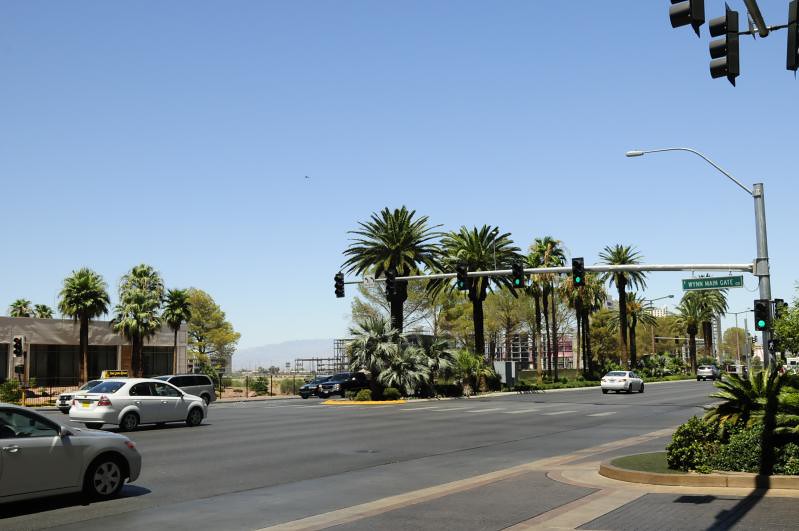This photograph captures a typical urban street scene. The road is flanked by curbs with plots of grass and bushes on either side. On the left side of the image, a row of palm trees stands tall. Behind these trees, there is a gray building partially obscured by the foliage, with three trees planted directly in front of it. 

On the road itself, a white car is positioned in front of the gray building, while a gray car is to the right of the white car. Overhead, a traffic pole extends across the street, holding a green traffic light. 

The street is a paved thoroughfare with various vehicles, including a white car that appears to have just passed through the intersection under the green light. The overall scene is a snapshot of daily life, with cars moving through a standard urban intersection.